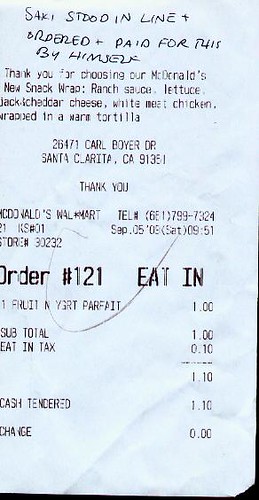This image is a photograph of a plain white receipt from McDonald's, featuring black text and a handwritten note at the top. The handwritten note reads, “Saki stood in line and ordered and paid for this by himself.” This seems to commemorate a personal milestone. Below the note, the receipt thanks the customer for choosing McDonald's new snack wrap, which includes ranch sauce, lettuce, jack cheddar cheese, and white meat chicken wrapped in a warm tortilla. The printed information further includes the address of the McDonald's location: 26471 Carl Boyer Drive, Santa Clarita, California, 91351, identified as being inside a Walmart. The actual order consists of one fruit and yogurt parfait, priced at $1.00, with a $0.10 eat-in tax, totaling $1.10. Order number 1218N is marked, with no change given from a cash tendered amount of $1.10.